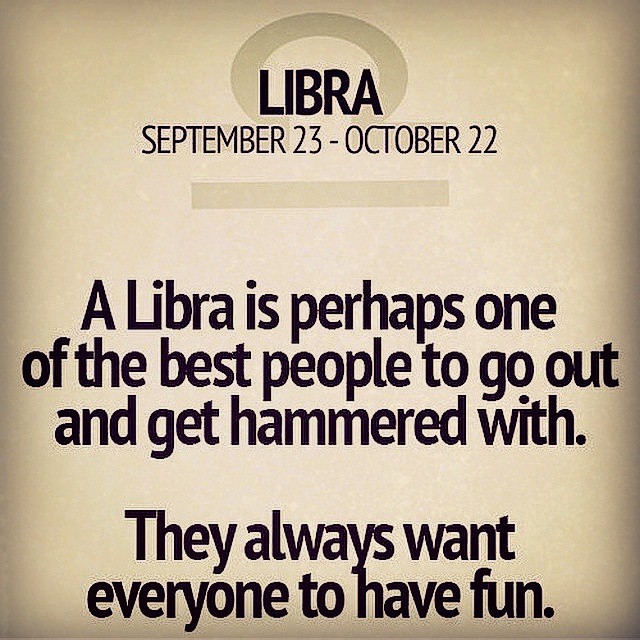The image features a sepia-toned background with a dark shading around the edges. At the top, in bold black uppercase letters, is the word "LIBRA," followed by the date range "September 23rd - October 22nd." Below this, there is an astrological symbol of Libra, consisting of a circle with a line underneath it. The text below reads, "A Libra is perhaps one of the best people to go out and get hammered with. They always want everyone to have fun." This description is written in black font over the sepia-toned background, emphasizing Libra's sociable and fun-loving nature.